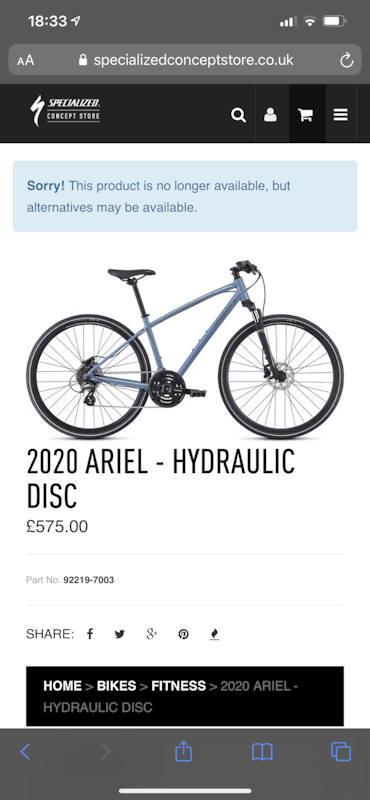A detailed caption for the image described would be:

---

The image showcases an e-commerce website displayed on a smartphone screen, specifically displaying the Specialized Concept Store at SpecializedConceptStore.co.uk. At the top of the smartphone screen, the time reads 18:33, with three bars indicating a strong signal and an almost full battery. The Specialized logo, featuring a stylized, swoosh-like vertical 'S' akin to Zorro's slashes, is prominently displayed next to various icons—search, user profile, shopping cart, and a hamburger menu.

Beneath the header, a blue notification banner addresses users with an error message: "Sorry! This product is no longer available. Alternatives may be available." The product in question is a 2020 Aerial Hydraulic Disc Mountain Bike priced at £575, identified by part number 92219-7003.

Further down, social media sharing options are provided, including icons for Facebook, Twitter, Google+, Pinterest, and an unidentifiable flame icon. Below these icons, a breadcrumb navigation trail shows the path taken: Home > Care > Bikes > Care > Fitness > Care > 2020 Aerial Hydraulic Disc.

At the bottom of the screen, there is a gray navigation menu with blue icons featuring various functions: a blue back arrow (highlighted as active), a grayed-out forward arrow (indicating no further navigation available), an up arrow, an open page icon, and a stacked square icon.

---

This caption provides a comprehensive and organized description of the image, detailing the various elements and features displayed on the smartphone screen.